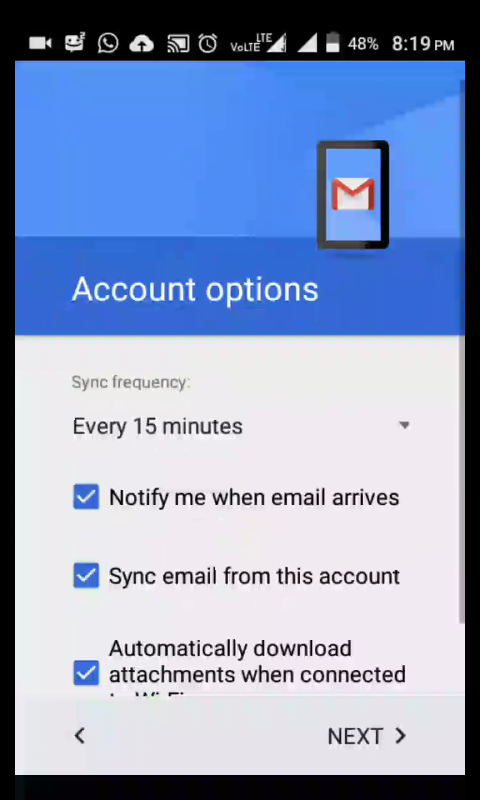In the image, likely a screenshot from a phone or tablet (judging by the aspect ratio and familiar icon indicators at the top), numerous details are captured. The status bar at the top displays the time as 8:19 PM, battery level at 48%, full wireless signal strength, an "LTL" signal indicator, and icons representative of a cloud, alarms, and notifications.

The main section of the screenshot is structured into distinct areas. At the top, a blue banner reads "Account Options" along with a Google Mail icon encased within a tablet graphic. Below this blue banner, a grey section contains several configurable options. The primary section is labeled “Sync frequency” and is set to "Every 15 minutes", accompanied by a toggle button.

Following this, there are three checkable options: “Notify me when email arrives” which is ticked in a blue box with a white checkmark, “Sync email from this account” also checked, and “Automatically download attachments when connected” marked similarly.

At the bottom of the screenshot, navigation buttons are visible: a forward button (pointing to the right) on the right side and a back button (pointing to the left) on the left side. Presenting this entire interface is a solid black border encapsulating the image.